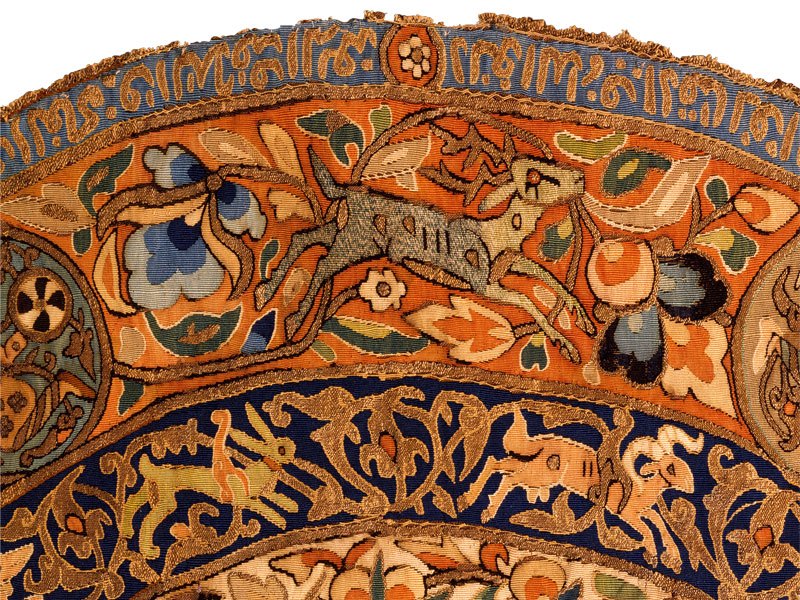This image shows a close-up of a portion of a decorative, vintage fabric that appears to be an ornate Oriental rug or tapestry, its edges showing signs of age and wear. In the center of this woven material is a detailed depiction of a deer or reindeer with dark body, brown head and neck, shown in mid-leap. Surrounding the deer is an intricate design of varying plants and flowers, with colors ranging from light to dark blue, light and dark greens with white edges, and leaves featuring orange centers and tan-like exteriors. The rug, primarily adorned in a blue and orange palette with beige trims, has ornamental vine patterns interwoven throughout. Also included in the design are multiple animals, including a white bunny with green body and long ears, and a ram or mountain goat with a light orange body, black lines, white-striped horns, and black-outlined eyes. The backdrop of the fabric is not visible, focusing the attention solely on the detailed and primitive art style of the intricate design.